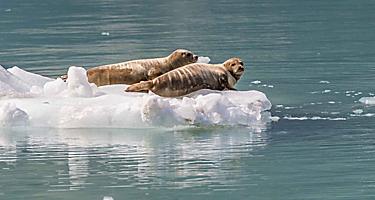The image captures a serene, natural setting during a bright day, featuring a group of light brown seals lounging lazily on a large ice floe. The scene includes a strip of white ice behind them, and the seals appear uninterested in their surroundings, epitomizing a sense of relaxed indifference. The vast ocean water beneath the ice floe is a grayish-blue hue, with tiny bits of cast-off ice floating around, suggesting a cold and pristine environment. The seals, appearing quite plump, are the focal point of this tranquil scene, showcasing the beauty and stillness of nature.